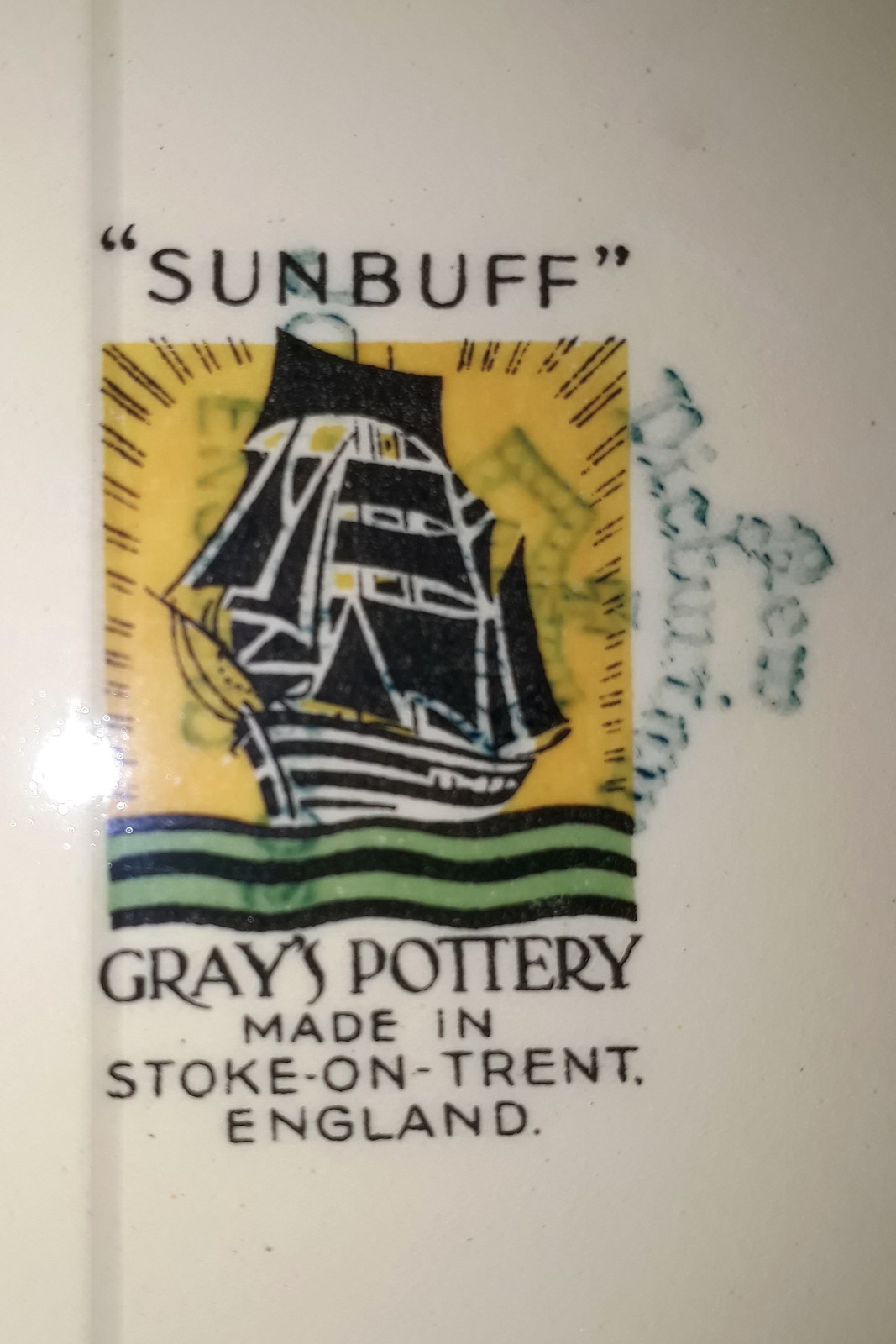The image depicts a detailed logo on what appears to be the underside of a piece of ceramic pottery. At the top, the word "sunbuff" is prominently displayed in quotation marks. Below this, a vibrant three-color illustration showcases a sailing ship with multiple black sails and black-and-white striped hull. The background features a yellow sky, green wavy patterns symbolize the water, interspersed with black stripes. Below the ship, the text "Gray's Pottery, made in Stoke-on-Trent, England" is clearly printed. Behind this image, a faint watermark or stamp is visible, adding an authentic touch to the overall design.